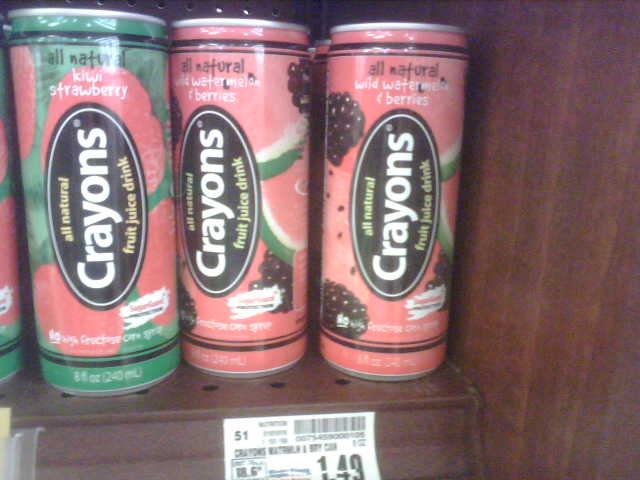This photograph captures an assortment of beverage cans positioned on a darker-toned wooden shelf. Below the neatly arranged cans, a price tag is visible, printed in black font. The image depicts two distinct flavors of beverages: Kiwi Strawberry and Wild Watermelon and Berries. The Kiwi Strawberry can features vibrant shades of green, pink, black, white, and yellow, while the Wild Watermelon and Berries can is adorned in light pink, black, white, and yellow hues. Each can proudly displays the label "All Natural Crayons Fruit Juice Drink" along with some additional white text near the bottom. Both cans are encircled with black rings near their top and bottom edges, adding a sleek touch to their design. The photograph itself appears somewhat blurry and has an aged quality, suggesting it might be an older capture.